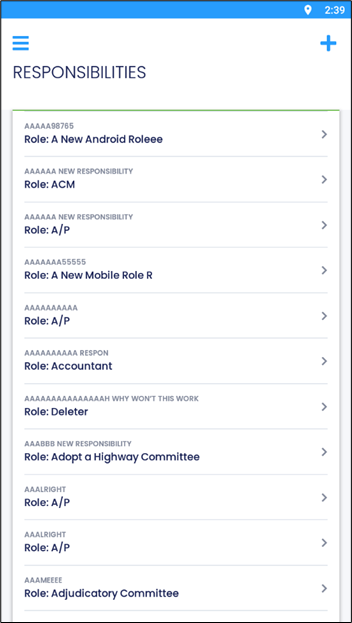A detailed caption for an image based on the given description:

"This image captures a screenshot from a mobile device, featuring a comprehensive list of responsibilities displayed on the screen. At the top of the screenshot, the title 'PRINT RESPONSIBILITIES' is prominently shown in bold, blue uppercase letters. Above this title, three horizontal lines on the left suggest the presence of a main menu that can be accessed via a dropdown, and on the right, a plus sign indicates the option to add new responsibilities.

Below the header, the screen is populated with a series of clickable menu items, each representing different roles. The first highlighted responsibility is labeled 'Role: New Android Role,' followed by other entries such as 'Role: ACM' and 'Role: AP,' all consistently displayed in bold, blue text. Interspersed among these roles are brief segments of text, seemingly marred by an overabundance of the letter 'A,' indicating possible typographic errors. Notably, there are candid comments such as 'Why won’t this work' within the text, suggesting frustration or additional notes.

The image overall portrays a digital interface for managing various roles and responsibilities within an application or system, providing users with multiple options for interaction."

This detailed caption provides a comprehensive understanding of the screenshot's content and context.